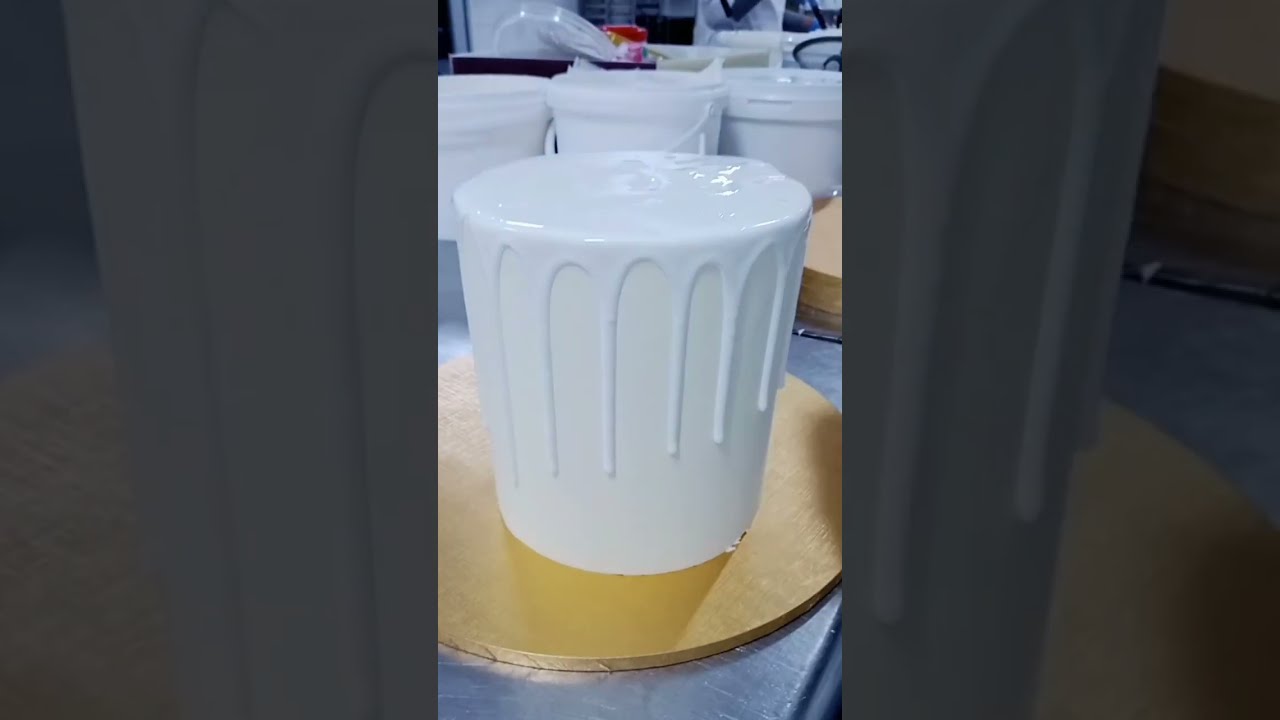This wide rectangular image features a central photograph of an overflowing white paint bucket. The bucket, placed on a golden wooden round surface, sits atop a light blue platform. Surrounding the central image are two close-up versions of the same scene, shaded much darker, located on the left and right sides of the image. The white paint is oozing evenly down the sides of the bucket, creating a pattern of lines. In the background, three additional white buckets can be seen, while a partially visible figure, dressed in white, seems to be manipulating objects and holding something red. The entire composition is uniformly framed in dark shades, giving a stark contrast to the brightly lit central subject.